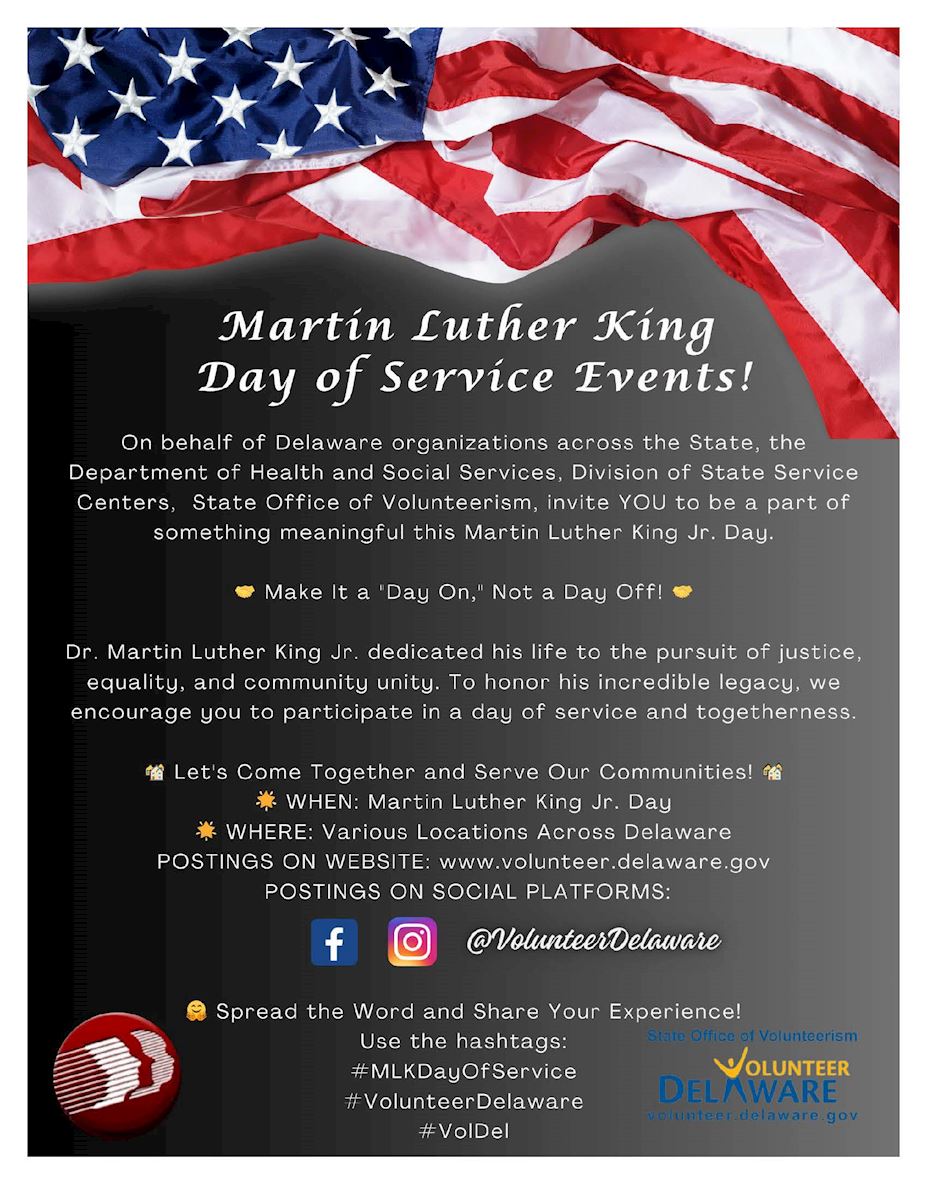The image is a detailed digital poster titled "Martin Luther King Day of Service Events." Dominating the top portion of the poster, a red, white, and blue American flag, slightly wrinkled, stretches from left to right. Below the flag, white text on a gradient background transitioning from super dark gray on the left to light gray on the right, reads: "Martin Luther King Day of Service Events!" 

A notable portion of the text says, "On behalf of Delaware organizations across the state, the Department of Health and Social Services Division of State Service Centers, State Office of Volunteerism invite you to be part of something meaningful this Martin Luther King Jr. Day. Make it a day on, not a day off." It also includes an inspirational quote: "Dr. Martin Luther King dedicated his life to the pursuit of justice, equality, and community unity. To honor his incredible legacy, we encourage you to participate in a day of service and togetherness. Let's come together and serve our communities. Spread the word and share your experience."

In the bottom right corner, there's the Volunteer Delaware logo in yellow and blue, followed by social media icons for Facebook and Instagram with the handle @VolunteerDelaware and hashtags such as #MLKDayOfService, #VolunteerDelaware, and #VolDell.